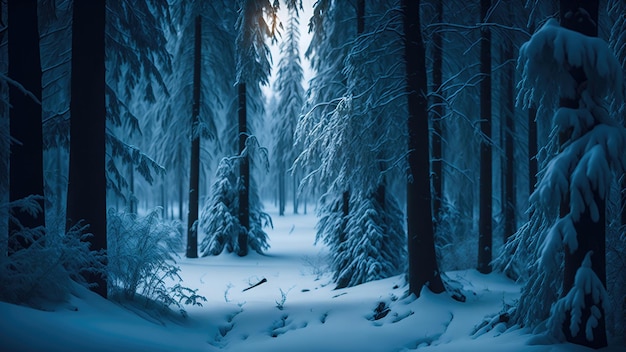This is an AI-generated, highly realistic painting of a snowy winter forest. The perspective is from a viewer standing in the midst of tall, dark-colored tree trunks, which are heavily laden with snow, causing their branches to bow towards the ground. Fir trees dominate the landscape, with numerous branches thickly blanketed in white. The forest appears to be thinly populated, providing a clear view through the trunks, yet still immersively wild and natural. In the center background, a singular, very tall, thin tree stands out, silhouetted against a bluish sky that is partially visible through the forest canopy. Sunlight filters gently, casting a lighter glow down the path that occupies the middle of the scene and revealing subtle animal footprints in the snow. Although the snow is generally white, shadows imbue certain areas with a bluish-white tint. Little bushes peek through the snow on the left side of the image, enhancing the serene and tranquil winter atmosphere.